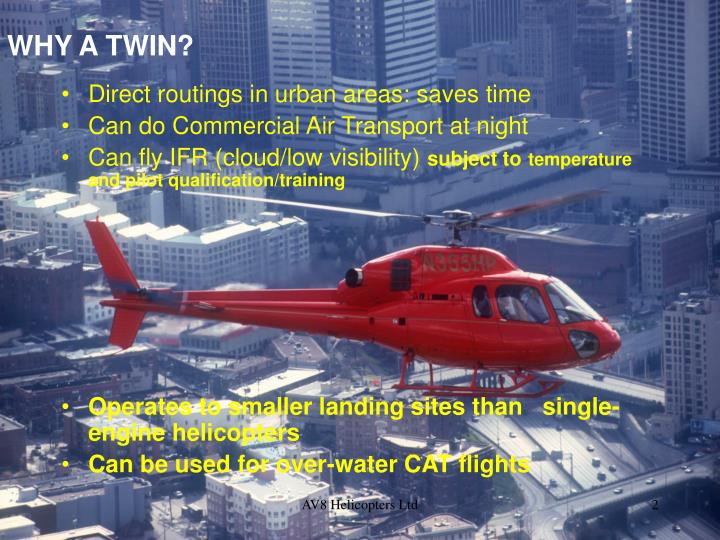The advertisement features a bright red twin-engine helicopter, centrally placed against an aerial view of a sprawling city with numerous tall buildings. The top left corner of the image includes white text reading "WHY A TWIN?". Beneath this heading are five yellow text bullet points: 

1. Direct routings in urban areas save time.
2. Can do commercial air transport at night.
3. Can fly IFR in cloud and low visibility conditions, subject to temperature and pilot qualification training.
4. Operates at smaller landing sites than single-engine helicopters.
5. Can be used for over-water CAT flights.

At the bottom of the image, in black text, it says "Aviate Helicopters Ltd."